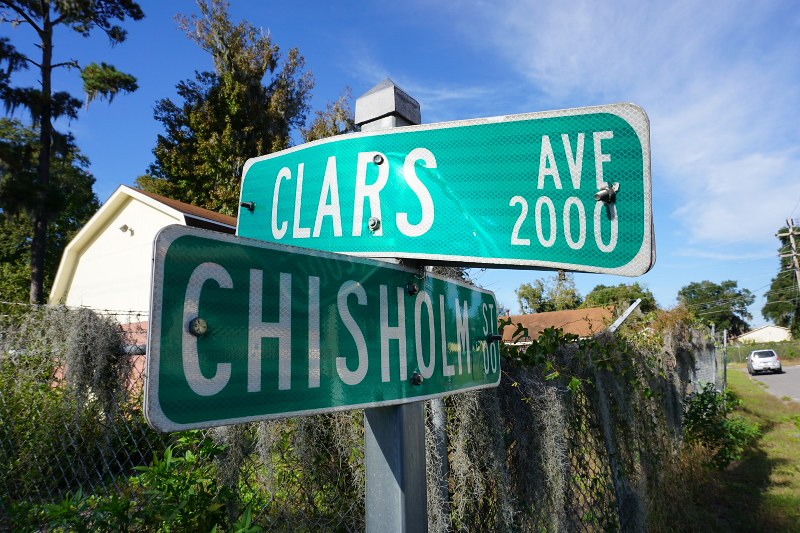The photograph captures a close-up of two intersecting street signs on a sunny day in a rural neighborhood. Dominating the center of the image, the signs are green with white capital lettering and bordered in silver-white. The top sign reads "St. Clairs Avenue 2000" (with the spelling correction noted as "C-L-A-R-S"), running horizontally from left to right, while the bottom sign, labeled "Chisholm Street 00," angles from the lower left corner towards the back. Mounted on a silver-gray post with a four-sided pointed cap, the signs gleam under the sunlight coming from the left. In the background, a weathered chain-link fence, partially obscured by vines and overgrowth, extends from the left corner almost to the right edge of the frame. Just behind the fence, a house with a gabled roof and a floodlight is visible. To the upper left, fully leafed deciduous trees add a splash of green to the blue sky adorned with wispy cirrus clouds. A silver car, parked on what appears to be a residential street, completes the tranquil neighborhood scene.